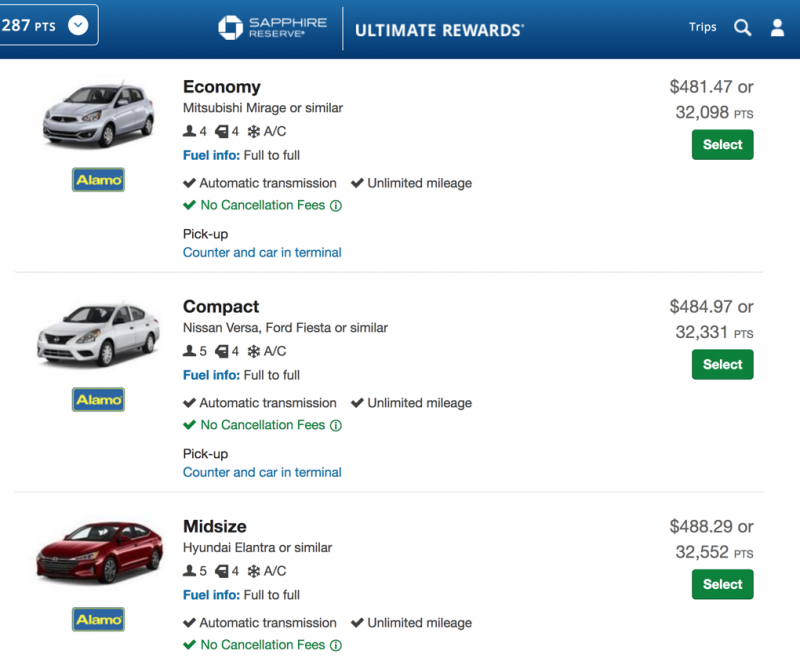This image shows a screenshot of a travel booking website. At the top, there's a blue banner. On the upper left side, the user's points are displayed as "287 points" with a pull-down arrow for more options. To the right, there's the "Sapphire Reserve" logo, followed by the text "Ultimate Rewards." In the upper right corner, there is a "Trips" link with a magnifying glass icon indicating a search bar.

Below the banner, set against a solid white background, a small silver car is prominently displayed. Below the car is the "Alamo" logo, which features yellow letters inside a blue box. To the right of the car, the text "Economy" is in bold, detailing that the car type is a "Mitsubishi Mirage or similar." The cost of renting this car is shown as "$481.47 or 32,098 points." 

Underneath the price, there's a green action button labeled "Select." Additional car information is provided below in blue and gray text, listing "Fuel Info" as "Full to Full" and confirming features like "Automatic Transmission" and "Unlimited Mileage" with a green check mark. Finally, the text "No Cancellation Fees" is highlighted in green.